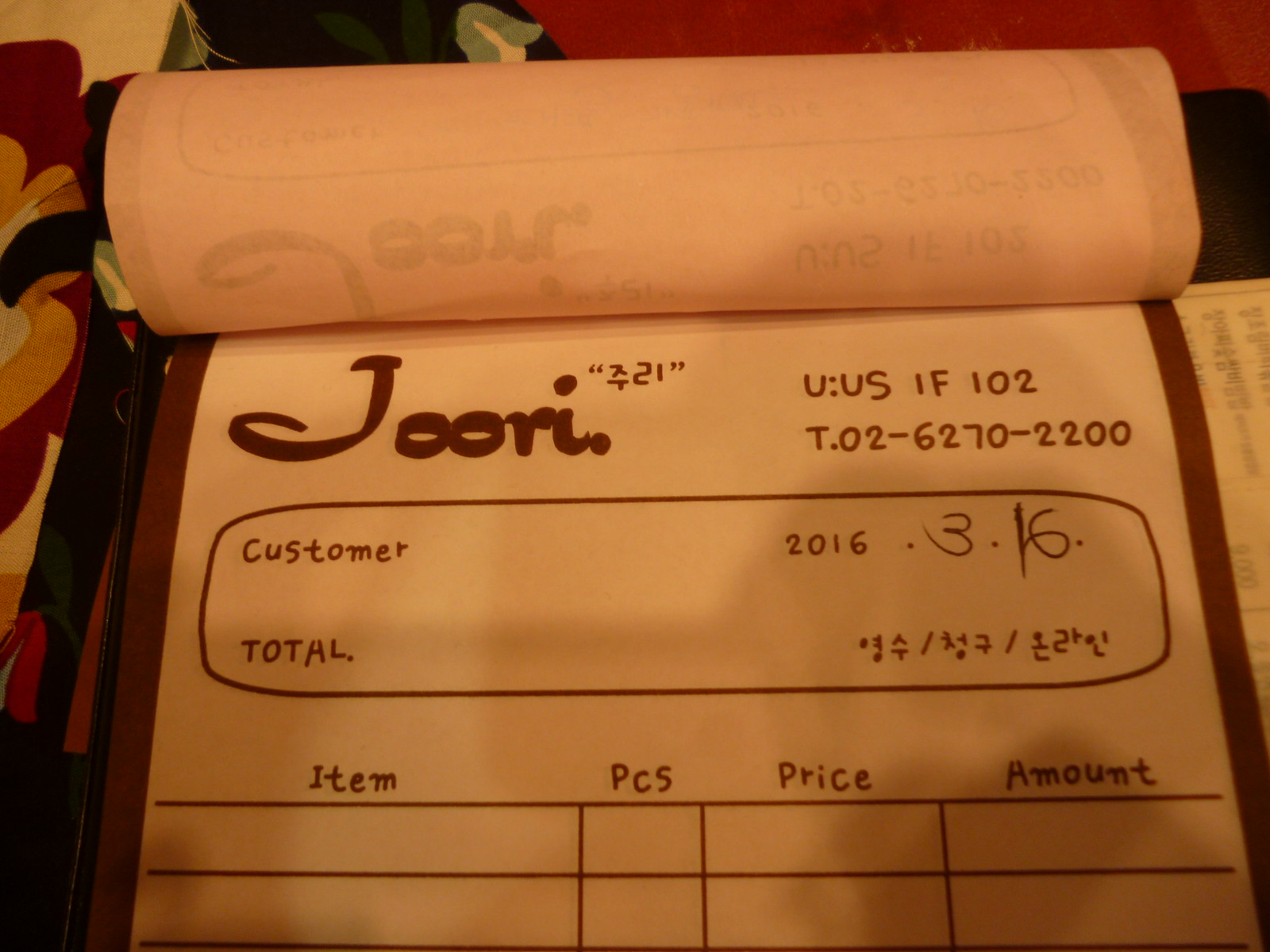A photo captures a small notepad from the store "Joori" (J-O-O-R-I), featuring a cursive or Middle Eastern-inspired font. At the top, there is partially discernible text indicating contact information ("telephone or U, U" followed by a string of numbers), whose exact purpose is unclear. Below this, the notepad includes columns labeled "Customer" and "Total," suggesting its use in a retail or food service setting, likely by a waitress or cashier. Further down, the sections "Item," "Pieces," "Price," and "Amount" are clearly outlined, indicating spaces for listing and calculating orders or purchases.